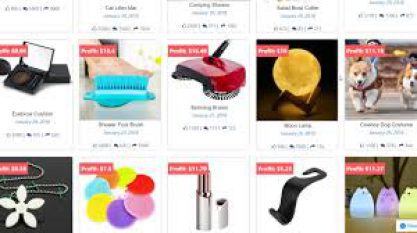This image is a screen capture from an unspecified shopping website, showcasing a series of blurred promotional items spread across two visible rows, each featuring indistinct red and white boxes, likely indicating special prices.

In the first row:
1. A black compact mirror.
2. A turquoise brush-like item.
3. A red and black metallic-looking device.
4. A lamp shaped like a yellow moon resting on a wooden surface.
5. An image of small tan and white corgis running.

In the second row:
1. A black square displaying a white flower necklace.
2. Several round, colorful objects in light blue, orange, yellow, red, pink, and purple.
3. A silver-colored tube of lipstick with the lid off.
4. A black wavy object with a hanging portion.
5. Abstract, light-up cat knickknacks in light blue, purple, and yellow-green colors.

The overall layout is somewhat blurry, preventing the exact identification of the promotional text or item names.